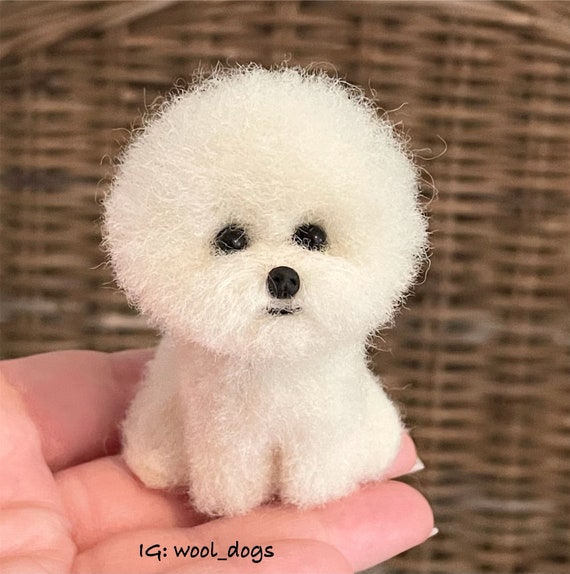In this close-up photograph, a tiny, adorable felted dog made entirely out of wool is prominently featured. The dog, resembling a cute little poodle puppy, is white, soft, and fluffy, with a noticeably large and round head. Its expressive face features two small black eyes, a button-like black nose, and a slight black line indicating a smiling mouth. The toy dog is in a sitting position with its four legs visible, giving it a charming and lifelike appearance. A woman's hand, visible from the left side of the image, delicately holds the woolen puppy against a wicker background, enhancing the cozy and artisanal aesthetic of the picture. At the bottom of the image, text reads "IG: wool_dogs," suggesting that this handcrafted creation is featured on the associated Instagram account.